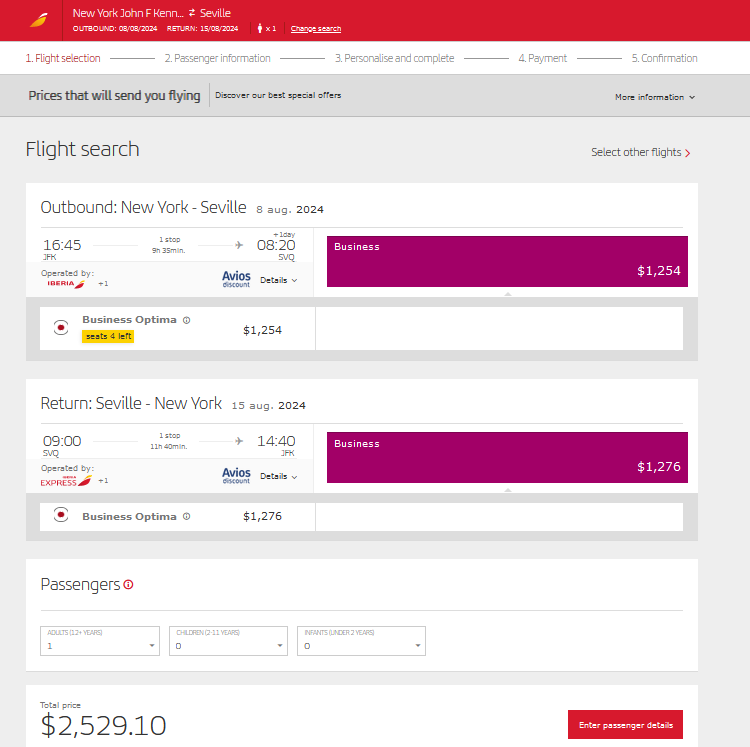### Screenshot of a Flight Booking Web Page

At the top of the web page, there is a prominent red bar. The top-left corner features a yellow and white symbol resembling a feather, which is the logo of Iberia Airlines. To the right of the logo, the text reads "New York John F K...," indicating John F. Kennedy Airport (JFK), followed by a right-pointing arrow and an airplane icon. The next entry reads "Seville SEB ILL E" indicating the destination. Below this, the flight details include: 

- Outbound: 08/08/2024
- Return: 15/08/2024

There is an icon of a person next to the text "1 adult," and "change search" is underlined. Below this is a sequence of numbered sections:

1. Flight Selection (highlighted in gray)
2. Passenger Information (separated by a gray line)
3. Personalise and Complete ("Personalise" with 's', separated by a gray line)
4. Payment (separated by a gray line)
5. Confirmation (separated by a gray line)

Under this sequence, there's a large gray box with a message: "Prices that will send you flying. Discover our best special offers." There is a "more information" drop-down and a "search other flights" option with a red arrow pointing to the right.

In the white box underneath "Flight Search," the outbound flight details are:

- Route: New York to Seville
- Date: 8 August 2024
- Departure: 16:45 from JFK
- Duration: 9 hours 35 minutes with one stop

A gray line under this has a small airplane icon followed by "plus one day 08:20 SBQ," indicating the arrival details. The outbound flight is operated by Iberia. To the right, there's an "Avios discount details" drop-down and a purple bar displaying the price: $1,254. 

The class selected is "Business Optima," marked with a red dot, and a yellow bar shows there are "seats for left."

The next white box provides the return flight details:

- Route: Seville to New York
- Date: 15 August 2024
- Departure: 09:00 from SBQ
- Duration: 11 hours 40 minutes with one stop
- Arrival: 14:40 (JFK)

This return flight is operated by Iberia Express. To the right, there's another "Avios discount details" drop-down and a price of $1,276.

Again, "Business Optima" is selected, marked with a red dot.

At the very bottom, under the "Passengers" section:

- Adults (12+ years): 1 selected
- Children (2-11 years): 0 selected
- Infants (under 2 years): 0 selected

The total price is $2,529.10, and a red bar at the bottom invites users to "Enter Passenger Details."